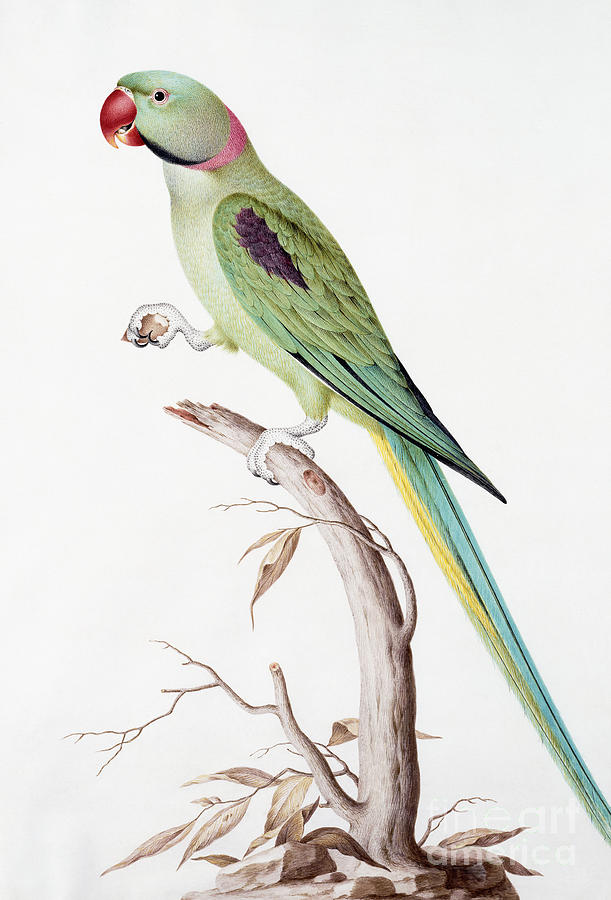This illustration depicts a ring-neck parakeet expertly rendered in a pen and ink sketch combined with watercolor. The background is stark white, accentuating the vivid subjects. A light tan tree branch, curving upward and to the right, occupies the lower half of the image and serves as the bird’s perch. The branch is adorned with brown, dry leaves at its base.

The parakeet, positioned in a side profile facing right, displays a dazzling array of colors. Its head and body are enveloped in a seafoam light green hue, with a distinctive pink band encircling its neck. The bird’s beak is a striking red. The feathers on its wings transition from light green to a deeper, almost turquoise blue towards the tips, with a small gray teardrop-shaped patch visible in the middle. The elongated feathers at the base of its wings exhibit this same blue hue.

The parakeet's long tail feathers mirror the turquoise blue of the wings, underscored by a layer of yellow that stretches the length of the tail. Notably, the bird’s claws are depicted with one gripping the branch and the other raised in mid-air, seemingly clasping an unseen object. The bird’s striking features and detailed feathers, combined with the simplicity of the white background, emphasize its vibrant and elegant appearance, capturing a superbly vivid and lifelike essence.